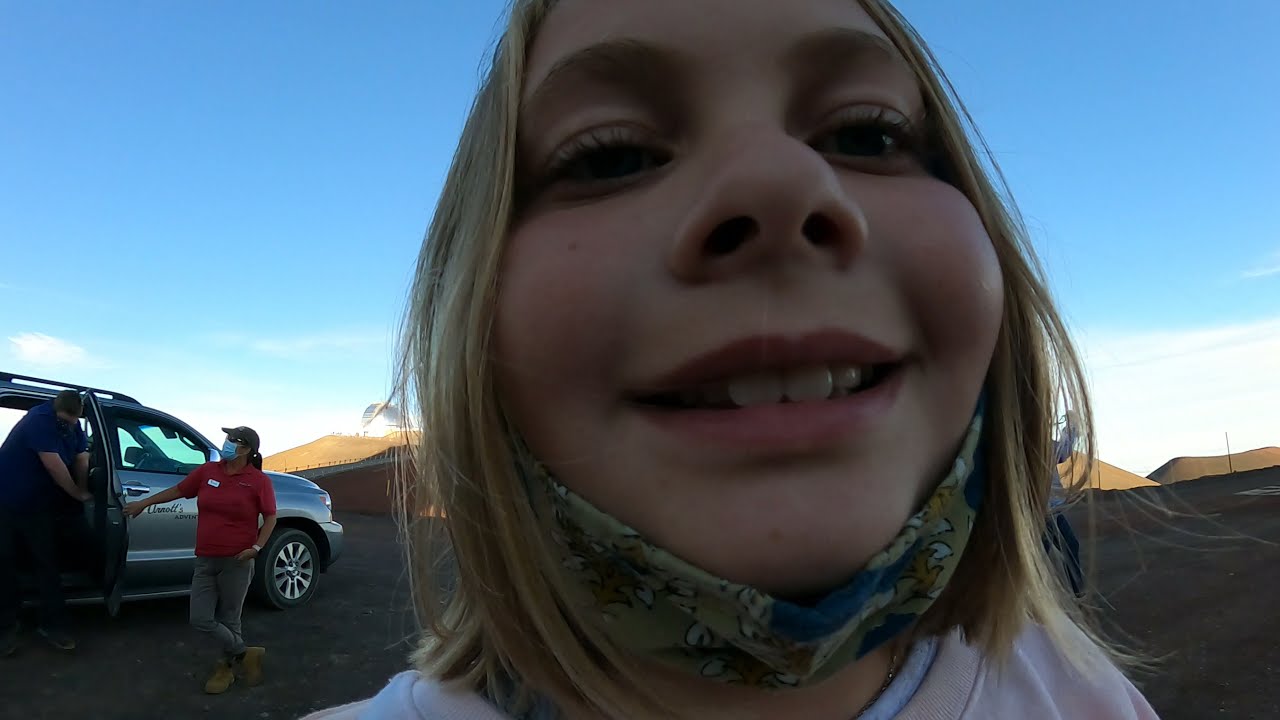This image features a young blonde girl, approximately 10 years old, taking a close-up selfie outdoors. She has peach skin and is smiling brightly, with a yellow, white, and blue mask hanging around her chin. She wears a white t-shirt. The majority of the image is filled with her face, capturing a joyful, candid moment. In the background, over her right shoulder, a woman wearing a red polo, gray pants, and tan boots is seen opening a silver minivan door for a man in a blue t-shirt. The setting appears to be a natural outdoor area, likely a park or a valley, with tan hills in the distance and a clear blue sky dotted with white clouds. The only discernible text in the image is "Arnott's Advent" on the side of the car, hinting at an advertisement for an adventure company. Despite the background elements, the focal point remains the girl's cheerful face, creating an impression of a spontaneous adventure snapshot.